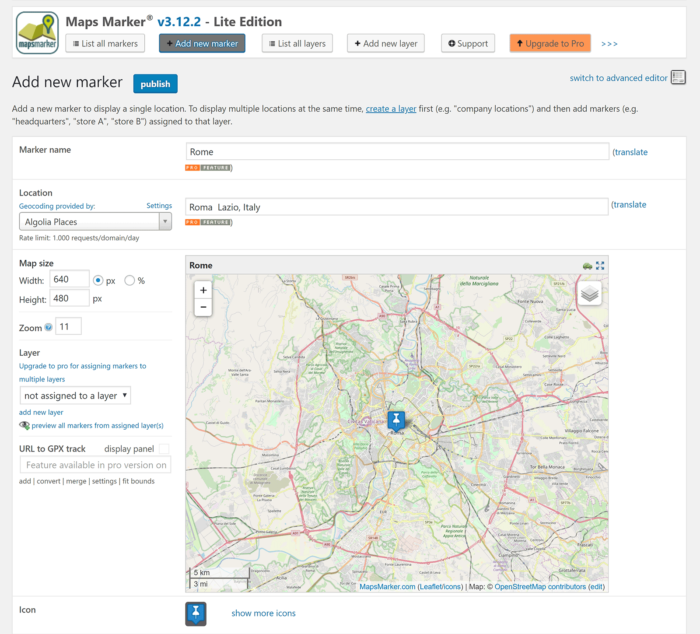In the top left corner of the interface, the text "Maps Marker" is displayed in a bold gray font. Adjacent to it on the upper right is a registered trademark symbol, followed by the text "v3.12.2" in blue, which indicates the version. To its right, a bold gray dash leads to "Light Edition," also in bold gray letters. 

Below this header, on the left side, there is a light gray, rectangular icon with a 3D appearance and a gray border. It features the text "List All Markers" along with three horizontal lines symbolizing a dropdown menu. Next to it, there is another rectangular icon with a medium gray background, showcasing a bold black plus sign and the text "Add New Marker" in light blue, bordered with light blue.

Continuing to the right, there are additional rectangular icons. The first one reads "List All Layers," followed by "Add New Layer," then "Support." Further right, there's an eye-catching orange icon with a bold upward-pointing arrow labeled "Upgrade to Pro," followed by three blue dots.

The background transitions to light gray below this section, where the workspace is divided into an interactive area. On the left side of this area, the heading "Add New Marker" appears in gray text. To the right, there is a blue rectangular button with the word "Publish" in white. Under this, gray text provides a brief instructional note: "Add a new marker to display a single location. To display multiple locations at the same time, create a layer." This statement includes a clickable link in blue and underlined text for more details. The instructions also include a parenthetical example: "(e.g., 'Company Locations')" followed by guidance on adding markers: "(e.g., 'Headquarters,' 'Store A,' 'Store B') assigned to that layer."